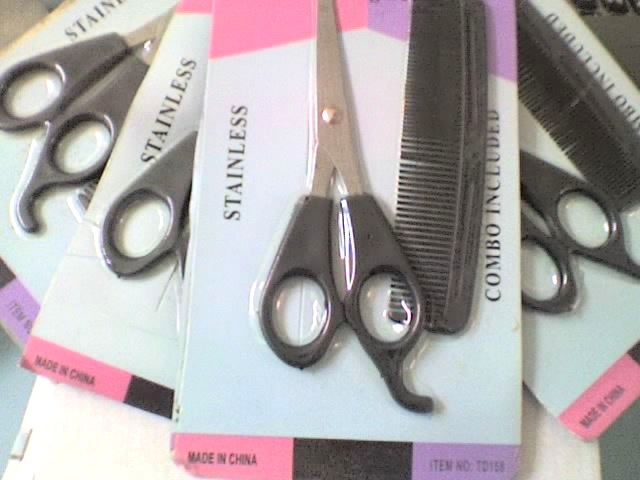The image depicts four unopened packages of hair-cutting scissors and black combs, each neatly arranged in a slightly fanned-out manner to display parts of each package. The topmost package is fully visible, showcasing a pair of stainless steel hair-cutting scissors with black handles alongside a black comb. The packaging is adorned with various labels: "stainless" on the left side and "combo included" on the right. At the bottom, "made in China" is printed on the lower left, and "item number 72158" is on the lower right. The packages themselves are colorful, featuring pink and purple hues with black elements. These sets appear intended for bulk sale or display in a shop.